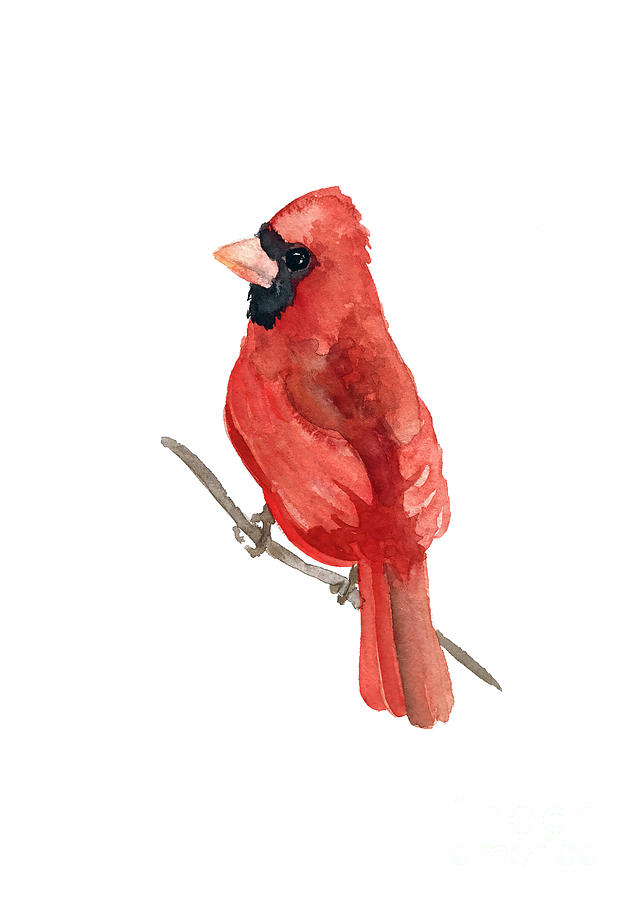The image depicts a watercolor painting of a male cardinal perched on a slender, leafless tree branch, facing to the left. The cardinal's body is predominantly a vibrant red, with a slightly darker red plume atop its head and along its back feathers. The wings exhibit a gradient transitioning to a lighter red, while the tips of the tail feathers show hints of brown. The bird's distinctive facial features include a small, triangular, pale reddish beak, framed by black markings that extend under its neck and around its shiny black eyes, providing a striking contrast against its red body. Brown claws are wrapped securely around the gray-brown branch, which is drawn with subtle detailing. Set against a plain white background, the simplicity of the painting accentuates the cardinal’s vivid coloration.